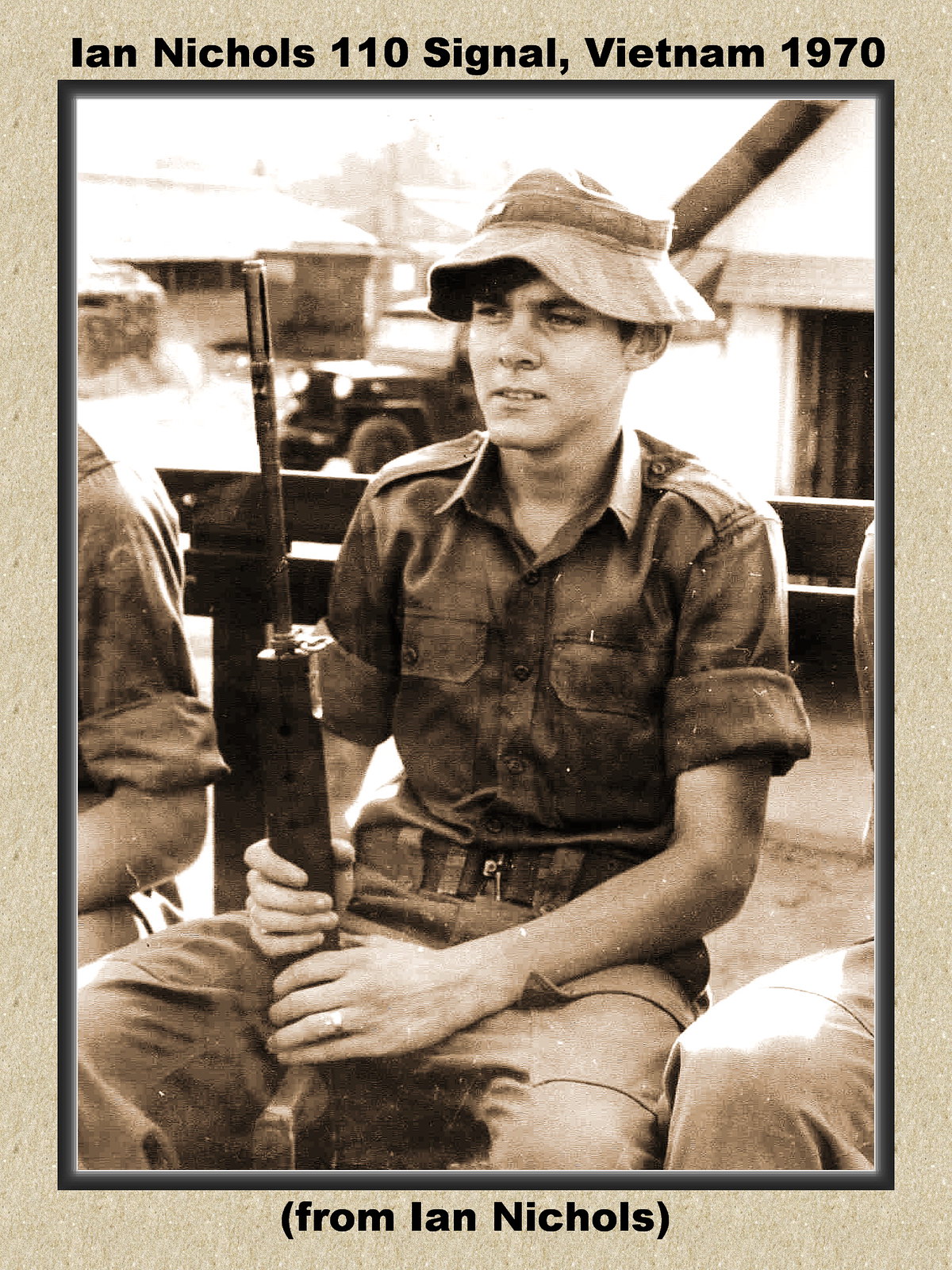In this black and white photograph titled "Ian Nichols, 110 Signal Vietnam 1970," a young soldier named Ian Nichols sits on a bench outdoors, holding a gun. The image, framed in black, also includes "(from Ian Nichols)" at the bottom, suggesting it was submitted for historical or wartime documentation. Nichols, dressed in a short-sleeved, collared uniform with rolled sleeves and standard-issue khakis, wears a bucket hat and appears to be looking slightly to his right, revealing a concerned yet neutral expression on his face. Behind him, a Jeep and a building with an open door are visible, along with the partial figures of two other soldiers—one to his left and the other to his right. The presence of these elements adds depth to the scene, evoking the everyday realities of soldiers' lives during the Vietnam War.